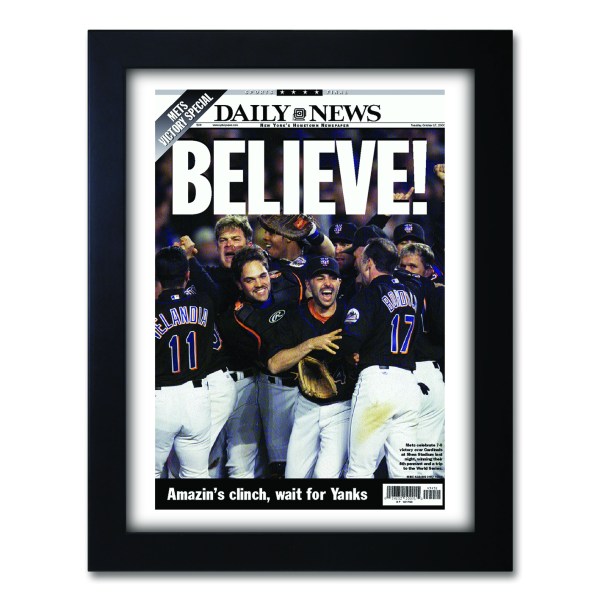The image depicts the cover of a Daily News magazine, encased within a photograph frame with a black border. The cover features a triumphant scene of New York Mets players, clad in their blue and orange uniforms with white pants, celebrating a recent victory. Their faces are lit with joy and excitement, capturing a raw moment of emotional exhilaration. The headline of the magazine prominently displays the word "Believe" in large white letters, underlined by the text "New York's Hometown Newspaper." A banner running along the side reads "Mets Victory Special," hinting at a championship triumph. Additional elements include smaller text and a barcode at the bottom, as well as a blurb stating "Amazing Clitch Wait for Yanks," likely related to the Mets' victory. The magazine cover, preserved within its black frame, suggests a moment from the early 2000s, immortalizing a significant triumph for the New York Mets baseball team.